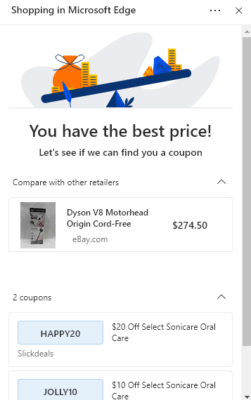This internet image showcases the "Shopping in Microsoft Edge" feature, highlighted at the top in a grayish-black font. The main visual depicts a blue-colored seesaw. On the left side of the seesaw, grounded, sits a large orange bag adorned with a black bow next to stacks of coins. On the elevated right side of the seesaw, there is a stack of coins and a blue triangle shape.

Beneath this image, the text reads, "You have the best price! Let's see if we can find you a coupon." Following this, there is a prompt to "Compare with other retailers" and a rectangular section displaying product information. It lists the "Dyson V8 Motorhead Origin Cord-Free" available on ebay.com for $274.50. To the left of this listing, a photo of the Dyson V8 Motorhead box is provided.

Further down, there's an announcement of two available coupons. The first coupon, enclosed in a white rectangular box, has a smaller light blue box labeled "HAPPY20," indicating $20 off select Sonicare Oral Care products, offered by Slickdeals. Adjacent to it, another rectangular box contains the "JOLLY10" light blue box, promising $10 off select Sonicare Oral Care items.